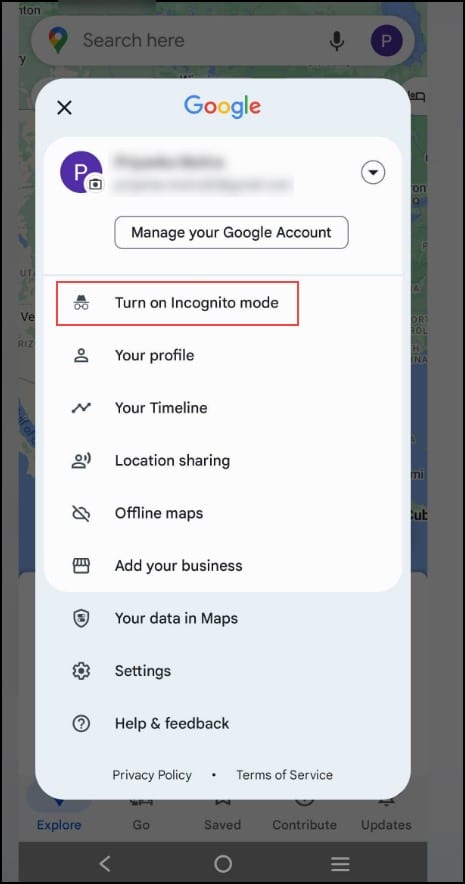The image depicts a screenshot of a Google search interface with a prominent pop-up window for account management. At the top of the screen, the iconic Google search bar is visible, featuring the multi-colored Google logo, a microphone icon, and a white 'P' inside a purple oval indicating a profile icon.

Beneath the search bar, a pop-up window with a light blue outline is displayed. This pop-up starts with the Google branding in its characteristic blue, red, yellow, blue, green, and red colors. Directly below this, another purple oval with the letter 'P' is shown, representing the user profile. Certain areas within the pop-up are grayed out for privacy and have a down arrow next to them. The pop-up prominently displays the text "Manage your Google Account."

In the pop-up, a list of options is presented. The first option, "Turn on Incognito Mode," is highlighted with a red rectangle around it, indicating it is selected. Other options include "Your Profile," "Your Timeline," "Location Sharing," "Offline Maps," and "Add Your Business." Further down, the background color transitions from white to blue, introducing additional options like "Your Data in Maps," "Settings," and "Help and Feedback." At the bottom of the pop-up, links for the "Privacy Policy" drop-down menu and "Terms of Service" are provided.

Below the pop-up window, the underlying screen can be seen with its main navigation options: "Explore," which is highlighted in blue, "Go," "Saved," "Contribute," and "Updates."

This detailed caption gives a comprehensive description of the screenshot's visual elements and interface functionality.